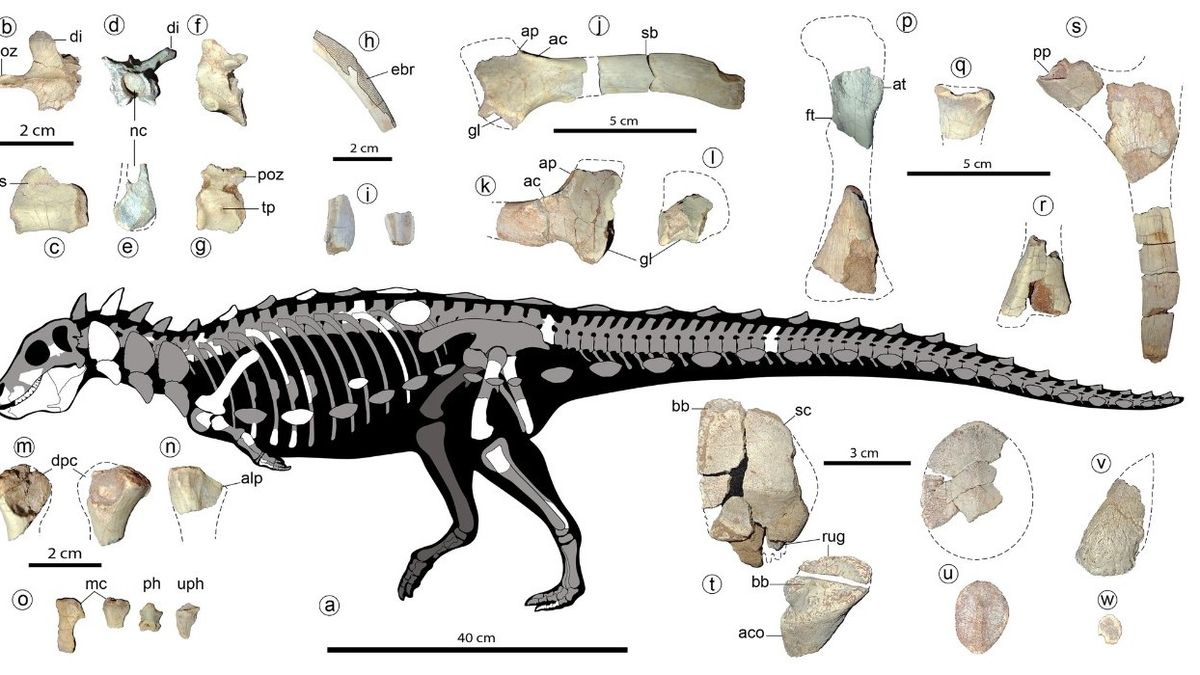The image is an anatomical chart of a dinosaur, displayed on a white background. At the center, there's a full-length, side-view drawing of the dinosaur's skeleton, rendered in shades of black, grey, and white. The skeleton prominently features regions highlighted in white, possibly indicating the actual fossilized bones that have been discovered. Surrounding the main skeletal diagram, there are various individual bones illustrated above and below the dinosaur. These bones vary in color, depicted in brownish, light blue, and grey hues, and are labeled with alphabets ranging from 'A' to 'W'. Each bone is accompanied by descriptive text that provides information and context about the bone's structure and significance. Additionally, dotted lines are used to outline the expected shapes of incomplete bones, offering a comprehensive view of the dinosaur's anatomy and emphasizing the piecemeal nature of paleontological reconstruction.